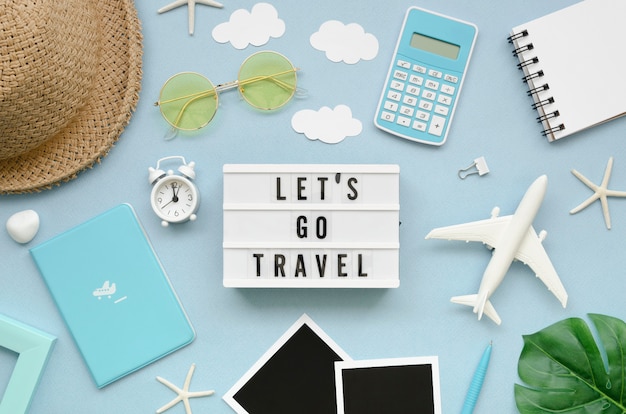The image depicts a collection of travel-themed items arranged on a blue table. Central to the composition is a plaque that reads "Let's Go Travel" in three lines of black text. Above this plaque, to the right, is a blue calculator, while to the left sits a pair of yellow-tinted round glasses. Directly to the right of the plaque is a small white toy airplane, and below it are two blank Polaroid pictures. On the left side is a small white alarm clock, next to a straw hat with a short brim that partially extends out of the frame. The bottom left corner features a white starfish, and the bottom right corner holds a green leaf. Scattered across the table are several cutouts, including white clouds and other decorative elements, enhancing the travel motif.